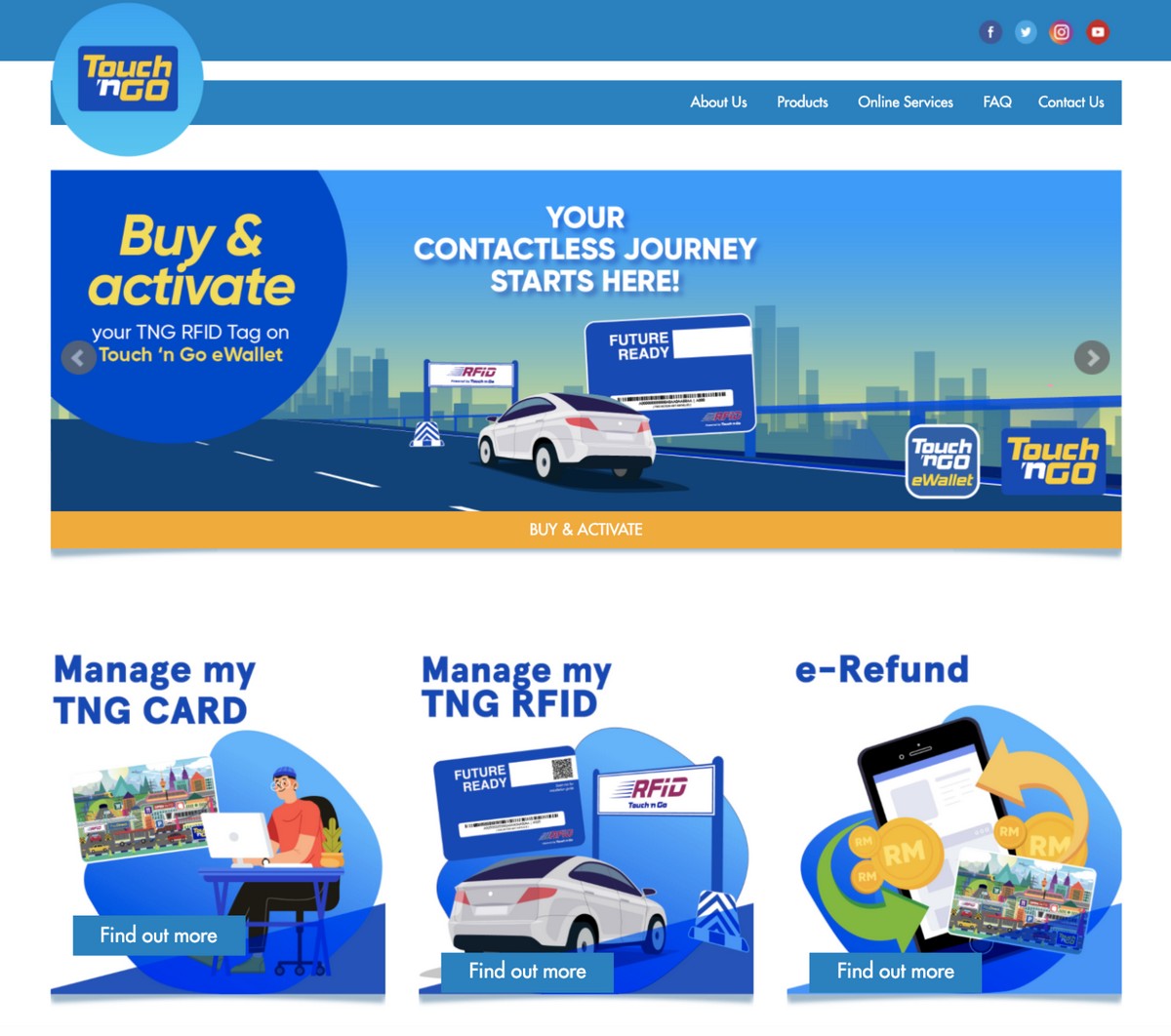This image features the homepage of the "Touch 'n Go" website. The logo, "Touch 'n Go," is displayed prominently with "Touch" and "Go" in yellow and an "N" in white. This text is set against a blue square with a light blue circle framing it. At the top of the page, there's a blue rectangular banner. In the top right corner, four social media icons appear in the following order: Facebook, Twitter, Instagram, and YouTube.

Below the banner, five navigation categories are displayed: "About Us," "Products," "Online Services," "FAQ," and "Contact Us," all in uppercase letters. Further down, an animated illustration captures a car driving down a blue highway. The background depicts a distant view of a city with skyscrapers against a blue sky.

On the left side of the image, the text reads "Buy and Activate" in gold. The main message in the center says, "Your TNG RFID tag on Touch 'n Go eWallet. Your contactless journey starts here." This is emphasized with an attention-grabbing yellow banner at the bottom that says "Buy and Activate" in white text.

Below this banner, three options are presented from left to right: "Manage My TNG Card," "Manage My TNG RFID," and "e-Refund." Each option is in blue text and accompanied by illustrative diagrams, all set against a white background at the very bottom of the page.